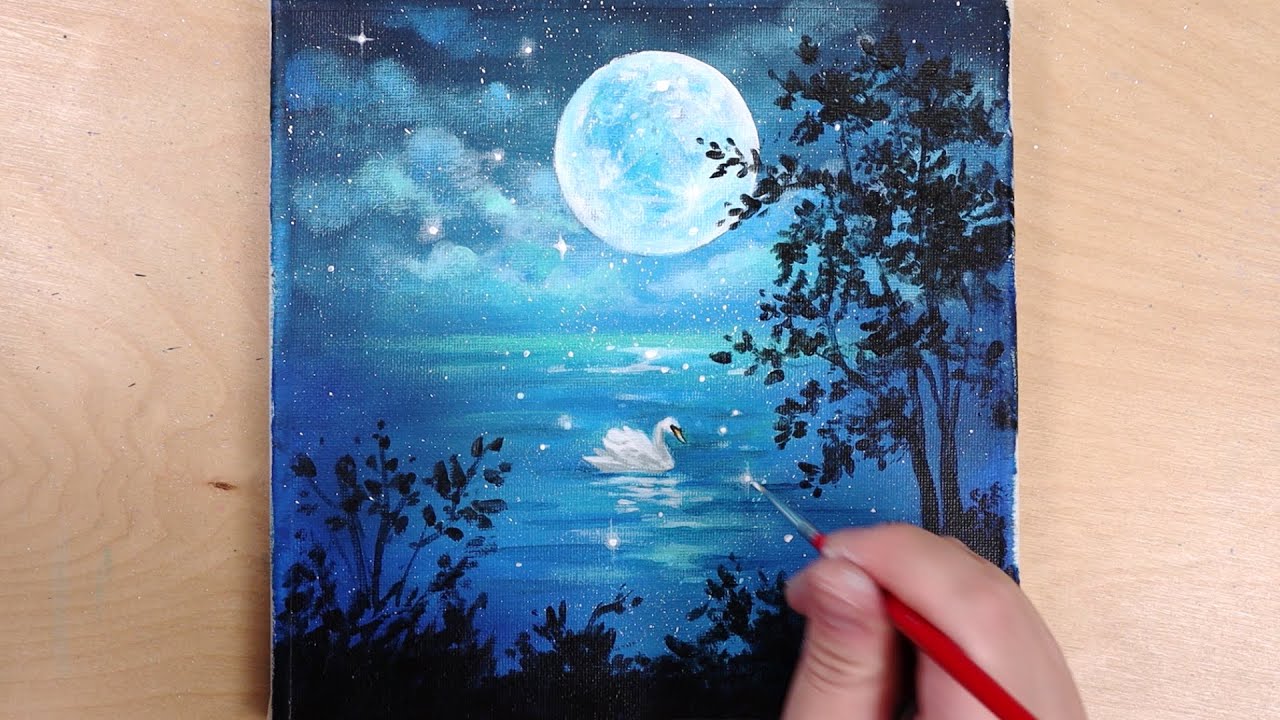In the overhead photograph, an artist is captured meticulously adding the finishing details to a small canvas painting, approximately the size of a stretched-out hand, with a red paintbrush. The canvas, resting on a light wooden table, depicts a serene night scene featuring a white swan gliding across a lake. The tranquil waters reflect the sparkling stars and a bright, full moon that casts a light blue hue across the scene. The background comprises various shades of dark blue, creating a night-time ambiance, while the foreground includes silhouettes of black trees, bushes, and leaves. Artfully rendered clouds in light blue hues hover above, adding depth to the nocturnal landscape. The painting, made using acrylic paints, showcases the artist's delicate brushwork as they bring this magical scene to life.